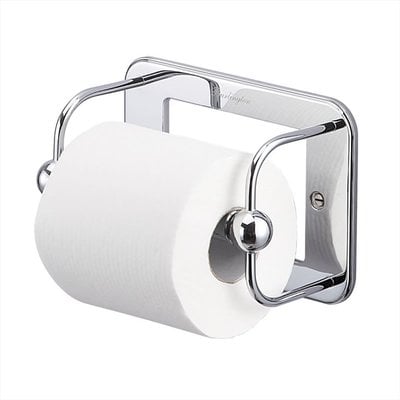The image showcases a distinctive silver, chrome-finished toilet paper holder mounted on a white wall. The holder features a unique rectangular design with a square cutout in the middle, lending it a modern, minimalist look. On the right-hand side of the holder, a visible flat head screw secures it to the wall. The holder’s arms curve downward and are capped with shiny round balls that keep the white toilet paper roll in place. The toilet paper itself is traditional white with a hollow cardboard tube in the center. The edges of the holder and its components are rounded, contributing to a sleek, polished appearance.